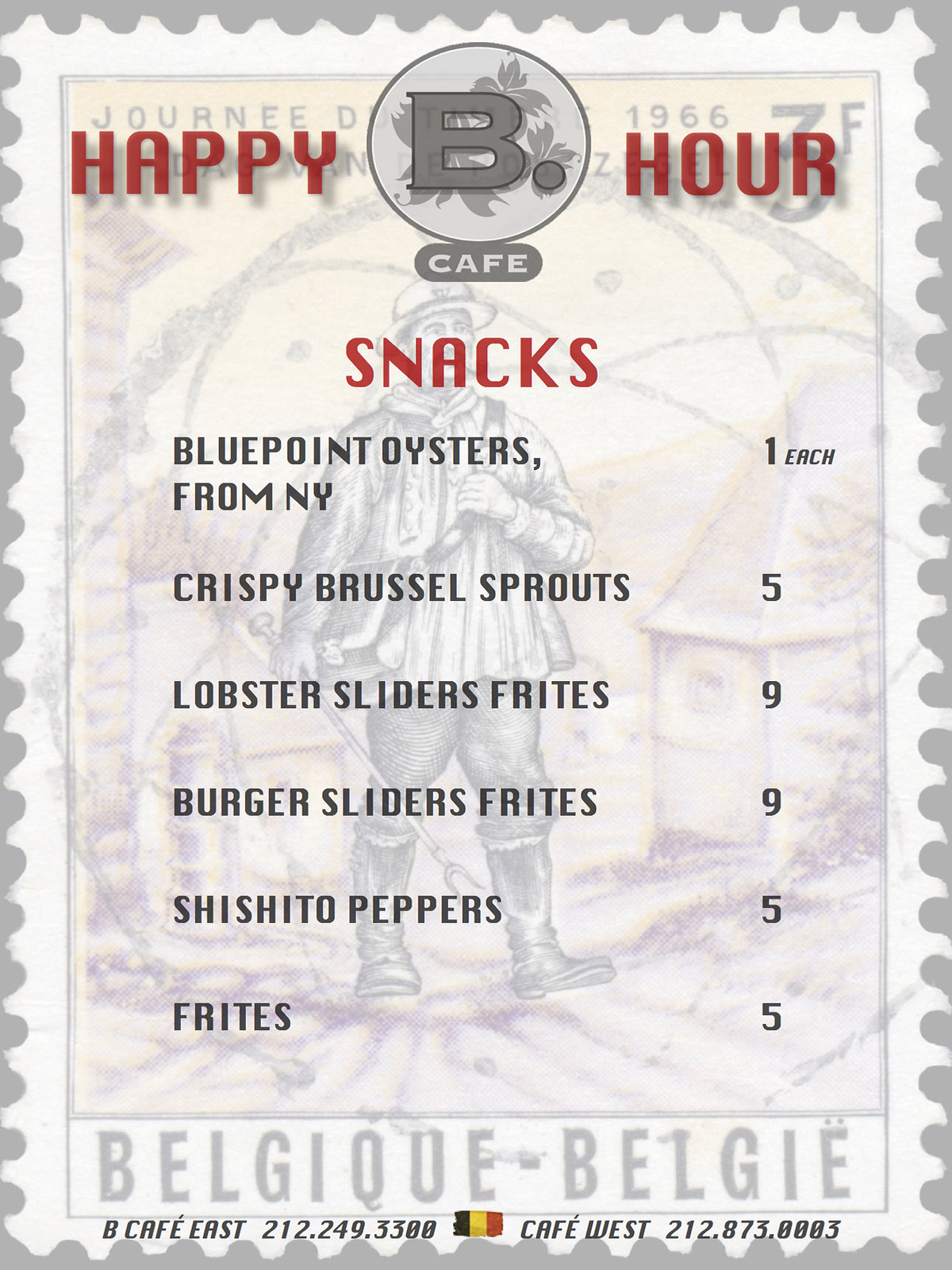The image showcases a "Happy Hour" menu from Happy Be Our Cafe. At the top of the menu, in bold red letters, it reads "Happy Hour" followed by "Snacks." The snacks listed include Blue Point oysters from New York ($1 each), Crispy Brussels sprouts ($5), Lobster sliders with frites ($9), Burger sliders with frites ($9), Shishito peppers ($5), and Frites ($5). Each item has its corresponding price clearly indicated.

The menu is set against a pale, almost translucent background featuring a drawing of a man. He appears to be wearing traditional countryside attire—including boots and holding a staff—and is walking across a rural landscape. Underneath this faint image, the words "Belgique" and "Belgi" are inscribed. At the bottom of the menu, the Belgian flag is displayed alongside the phone numbers for both units of Happy Be Our Cafe, labeled as "B Cafe East" and "Cafe West."